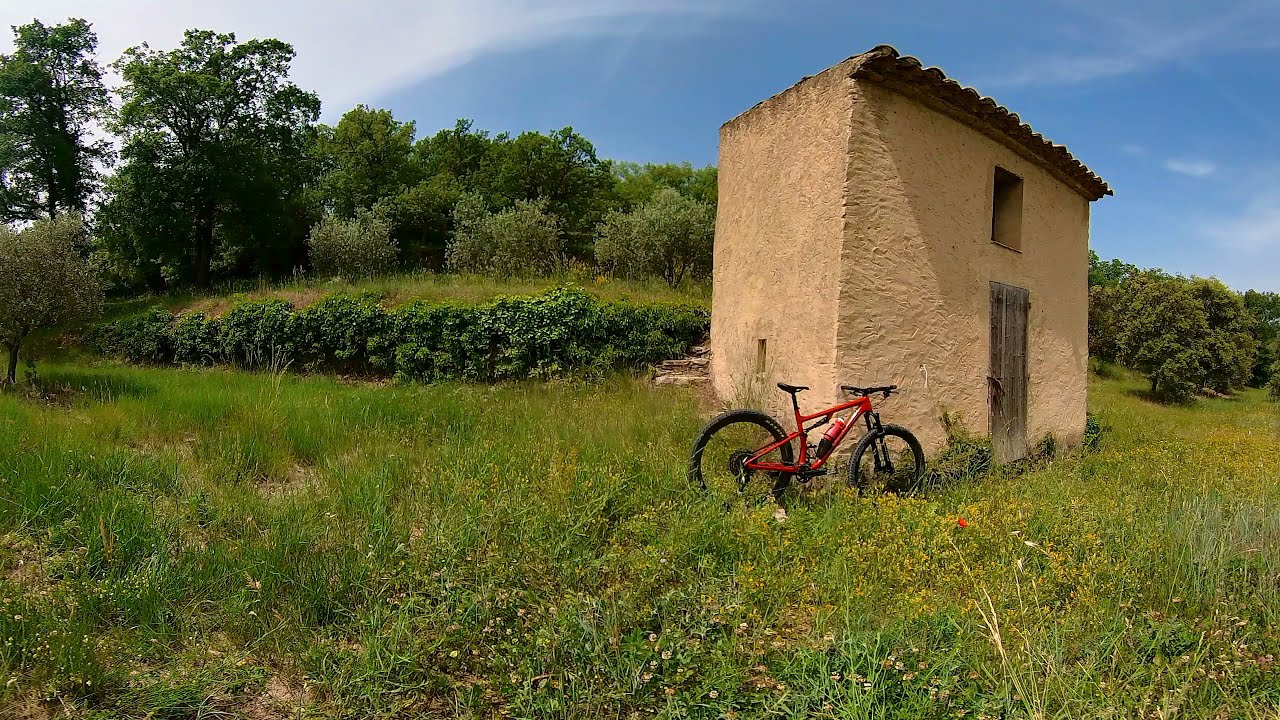In this outdoor scene, a small, stucco outbuilding with a worn wooden door stands prominently in the foreground. The building, likely a one-room structure, is a beige color with a tightly inset window on the left side and a larger window above the door on the right. Leaning against the building is a red and black mountain bike. The setting is a grassy field dotted with clumps of flowers, featuring a gentle incline that reveals a low wall of shrubbery and a backdrop of taller trees, suggesting a forested area. The sky above is blue with patches of white clouds, highlighting a clear, daytime atmosphere. This serene countryside image showcases a variety of colors including different shades of green from the grass and trees, the red and black of the bike, and the earthy tones of the outbuilding.